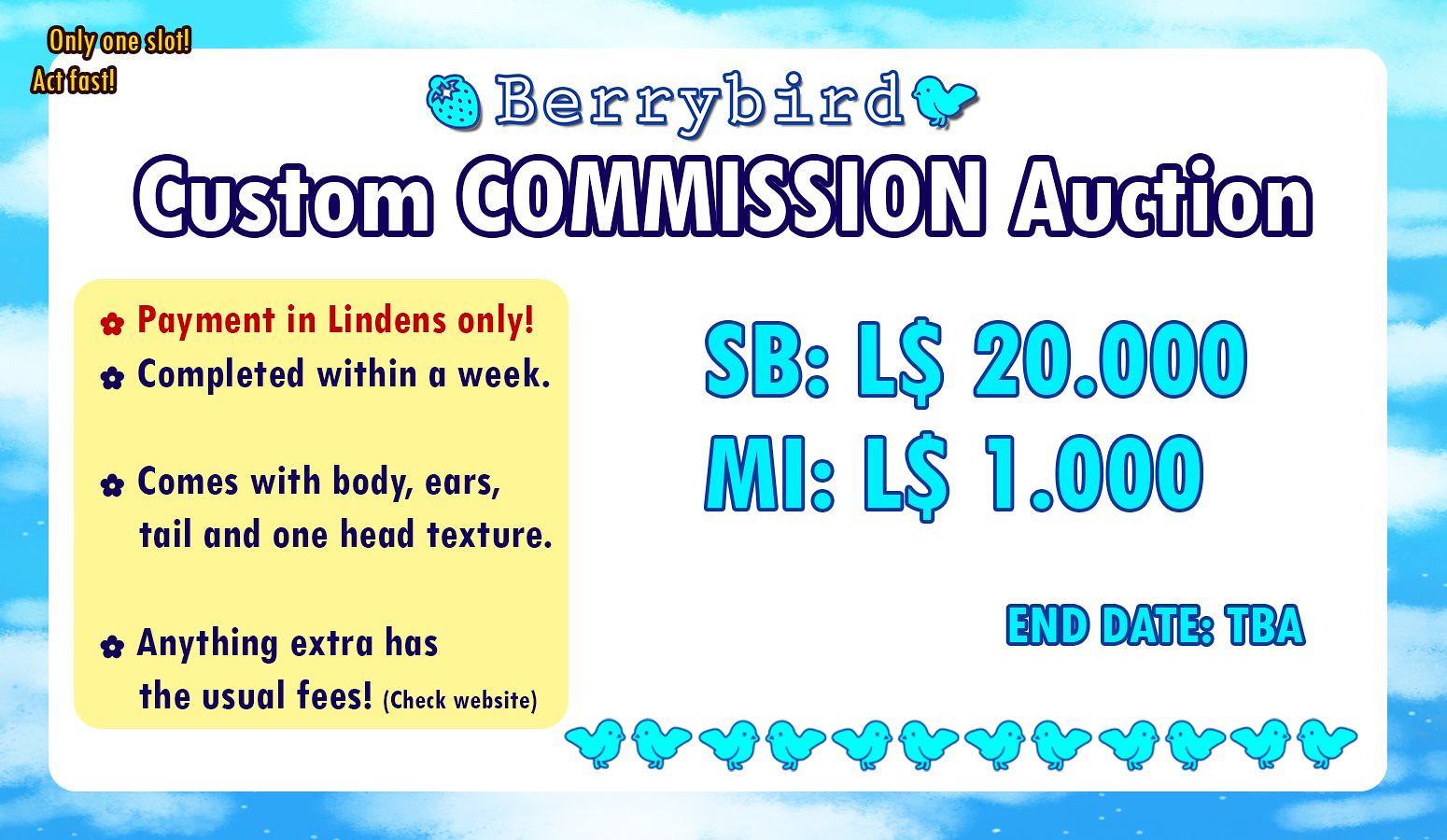The image is a detailed poster for a "Barry Bird Custom Commission Auction." The main background is white with a blue sky-like border filled with clouds. At the top-left corner, in bold yellow text outlined in black, it says, "Only one slot! Act fast!"

Centered at the top of the poster in white text with a blue outline is the title, "Berry Bird." Adjacent to the title, on the left, is an image of a blue strawberry, and on the right, a small blue bird. Below this, still within the central white area, the poster continues with the text "Custom Commission Auction" in outlined letters.

The left section of the poster features a yellow box containing the text in different colors. The red text reads, "Payment in Lindens only." Below this, in blue text, it says, "Completed within a week, comes with body, ears, tail, and one head texture. Anything extra has the usual fees (check website)."

On the right side of the poster, in blue text against the white background, it reads, "SB: L$20,000, MI: L$1,000, End Date: TBA." Along the bottom of the poster, there are several pictures of blue-colored birds, matching the one next to the title.